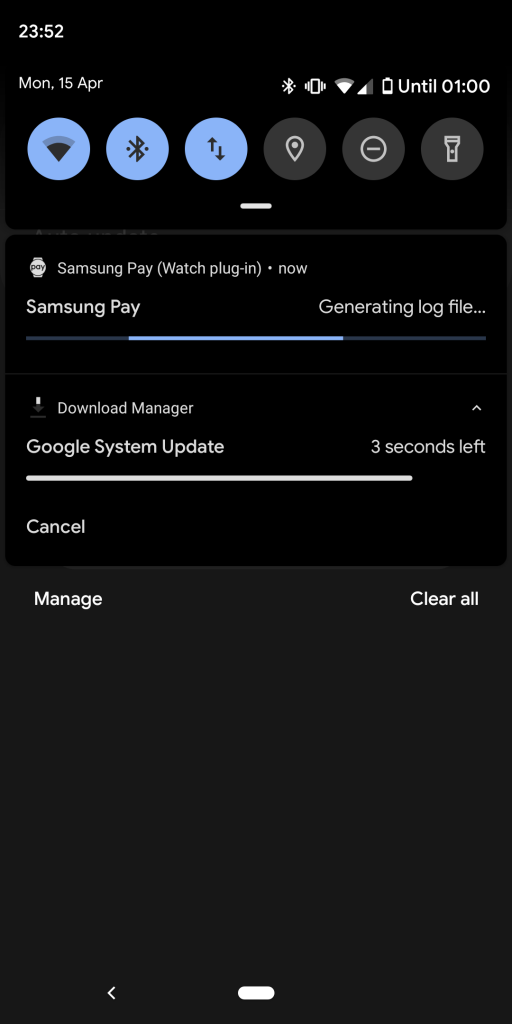The image depicts a long, vertical box set against a black background. In the upper left corner, the time is displayed as 23:52. Directly below the time, the date is shown as MON, 15th April. Adjacent to these details, on the right, are icons for a speaker and a battery. The battery icon is nearly empty, showing only a small white segment at the bottom, indicating it will deplete by 01:00.

Descending the screen, there are three blue circles followed by three gray circles, separated by a tiny white line. The subsequent row contains the text "Samsung Pay (watch plug-in), now." To the left of this text is "Samsung Pay" accompanied by a long blue line, and to the right, the phrase "generating log file."

Next in line is "Download Manager," followed by "Google System Update," which is highlighted by a lengthy white line underneath it. Just above the end of this white line, the text "three seconds left" is displayed. Moving further down, the word "cancel" is visible. About two inches below "cancel" is the word "manage" in white text, and approximately three inches to the right of "manage" are the words "clear all," also in white.